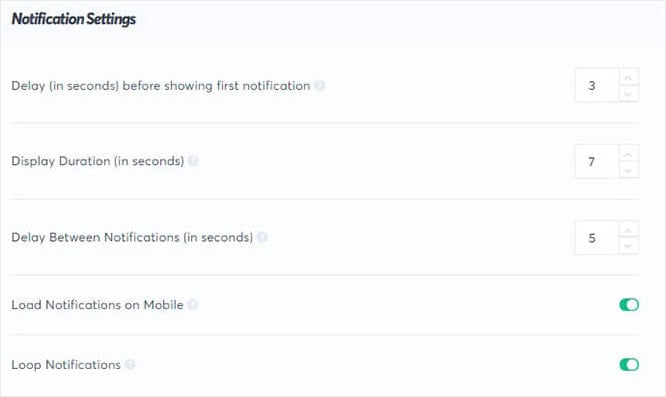This is a detailed screenshot of a notification settings dialog box.

The dialog box features a light gray background with a slightly darker gray outline. Across the top-left corner, "Notification Settings" is prominently displayed in bold and italicized black text. 

Below this heading, the first setting option reads "Delay (in seconds before showing first notification)" followed by a small, two-tone gray arrow (or possibly a question mark) to the right. Adjacent to this, a selection box shows the number 3, with up and down arrows available for adjusting the value.

The next option reads "Display Duration (in seconds)," again accompanied by the same two-tone gray icon to the right. Next to this setting, a box displays the number 7, also with adjustable up and down arrows.

Following this, the "Delay Between Notifications (in seconds)" option is similarly formatted with the gray arrow/question mark to the right and a selection box showing the number 5, complete with its up and down arrows for modification.

Further down, the "Load Notifications on Mobile" setting appears with the familiar gray arrow icon next to it. To the right, a rectangular toggle switch with rounded edges is displayed in green, indicating that this option is currently enabled.

The final setting, "Loop Notifications," follows the same layout with the gray arrow/question mark to its right and another green toggle switch on its right side, indicating it is also enabled.

Each setting is separated by a gray line that matches the dialog box's border, providing a clear visual distinction between the different options.